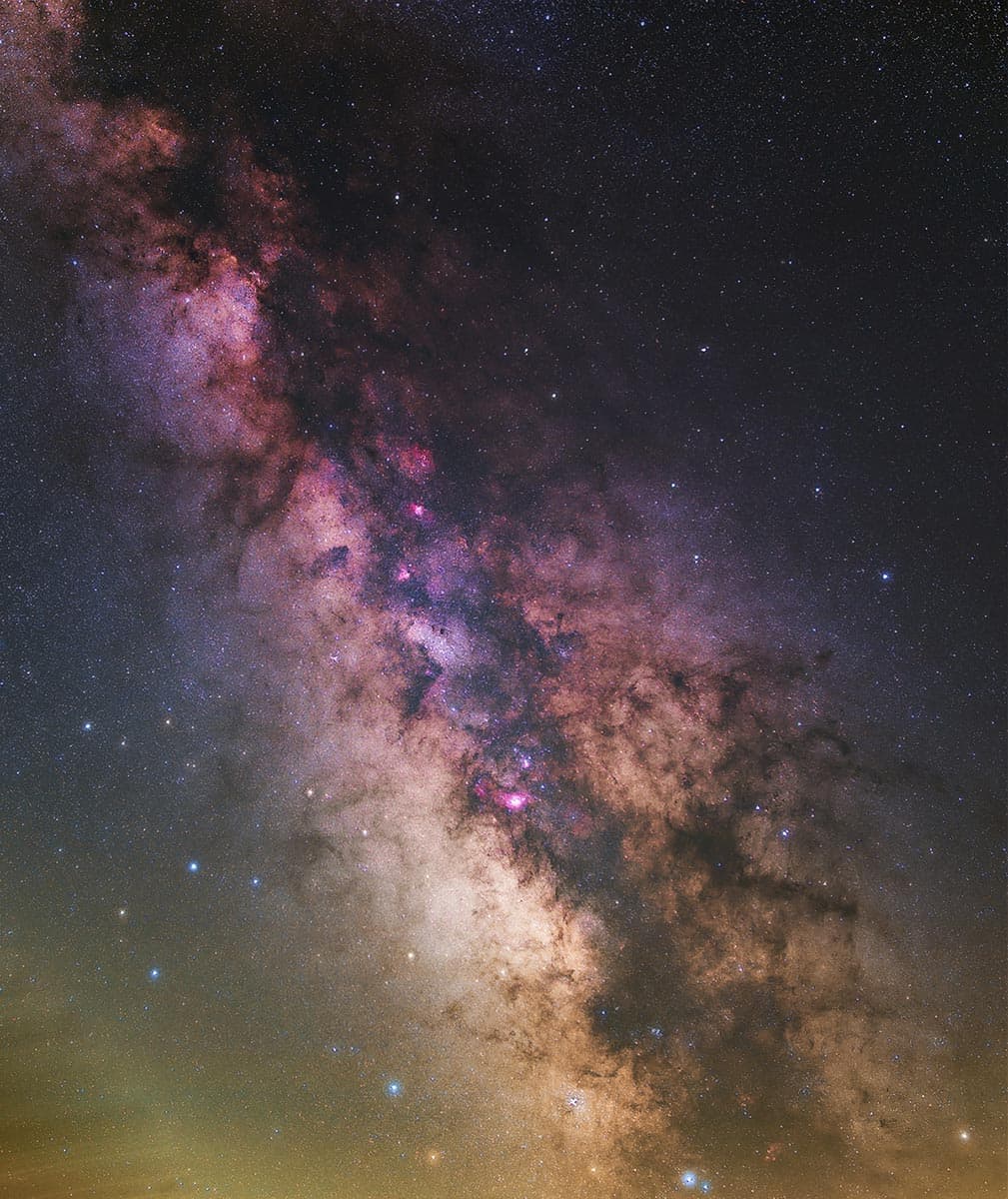This close-up image of outer space vividly displays a mesmerizing blend of colors and star formations. Dominating the top corner is a dark blue shade speckled with numerous tiny stars. The image transitions into a central area shrouded in dark, cloudy matter that almost resembles smoke or a storm cloud, a striking diagonal stretch of purples and blacks accentuating the mysterious beauty. To the left, the image lightens to a softer blue, adorned with brilliant, bright stars in varying hues of pink, orange, blue, and white. The bottom portion reveals a touch of gold, contributing to the overall captivating palette of the night sky. This beautiful cosmic vista not only highlights the dramatic contrast between different regions but also underscores the visual splendor of the stars, some appearing brighter and larger against the contrasting backgrounds.